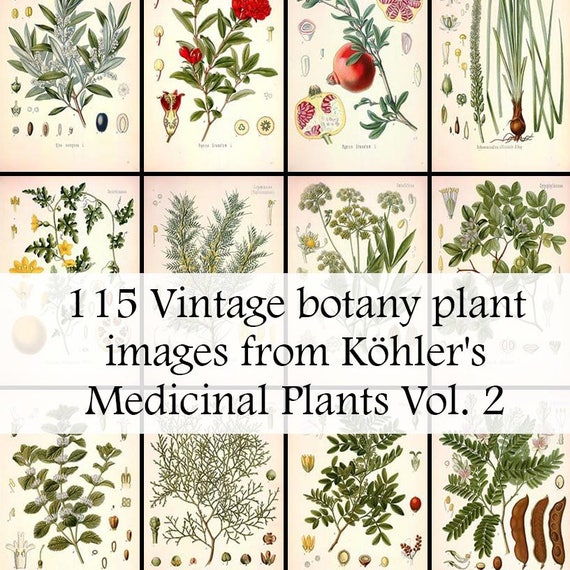This image features the cover of a vintage botanical book titled "115 Vintage Botany Plant Images from Kohler's Medicinal Plants, Volume 2." The cover is a detailed collage composed of twelve individual frames, neatly arranged in three rows of four. Each frame showcases a different plant species, meticulously illustrated, highlighting the book's scientific nature. The plants include a variety of herbs, flowers, fruits, and vegetables, such as an olive branch, chives, a pomegranate, and several medicinal herbs. The background of each frame is a faded ivory, underscoring the book’s vintage origin. Across the lower half of the cover, a translucent white strap prominently displays the title text. The image palette consists predominantly of greens, with vibrant accents of yellow, red, and brown, enhancing the botanical diversity depicted.